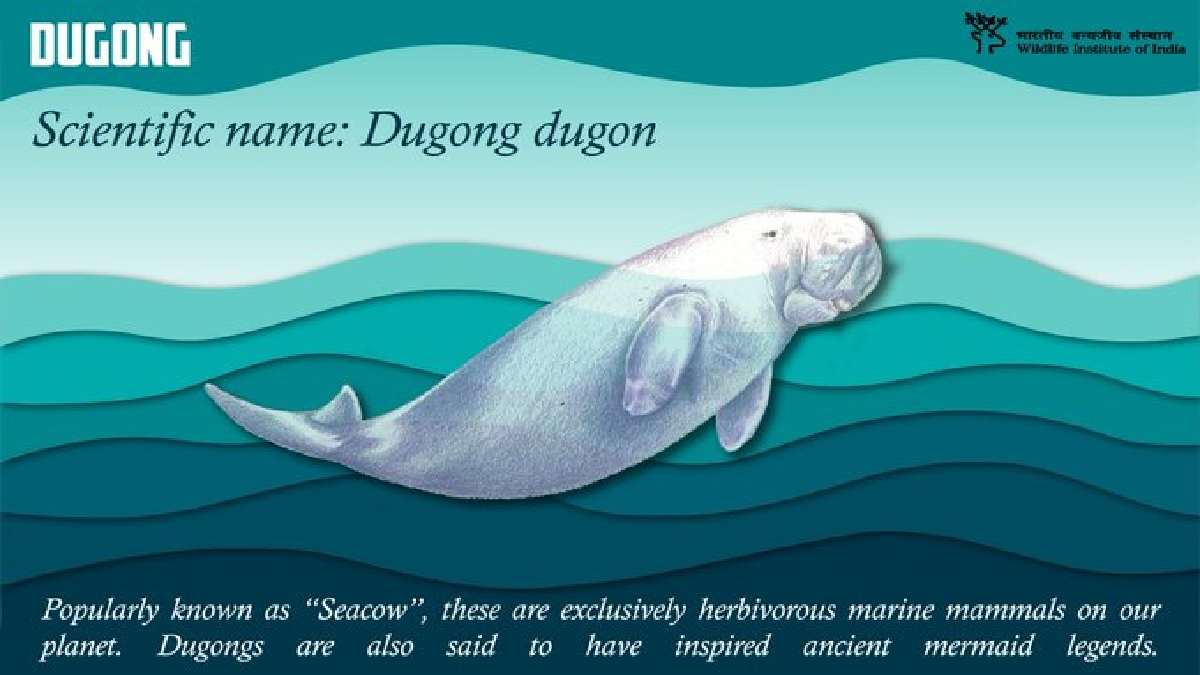The image is a detailed, illustrated poster of a marine mammal known as a dugong, prominently displayed in the center. The background features wavy lines and gradient shades of blue, transitioning from darker hues at the bottom to lighter ones at the top, evoking an underwater scene. In the upper left-hand corner, in white letters, it reads "DUGONG." Just below, it states the scientific name as "Dugong dugon." The central dugong illustration displays a grayish-white color with noticeable fins and a distinctively flat, smashed-looking nose or mouth area, with one eye visible on the right side of its face. The dugong's slightly curved tail fin can be seen, hinting at the mermaid legends it supposedly inspired. At the bottom of the image, white text explains: "Popularly known as the sea cow, these are exclusively herbivorous marine mammals on our planet. Dugongs are also said to have inspired ancient mermaid legends." In the upper right-hand corner, there is a blurred logo including the words "Wildlife Institute," possibly "of India." The overall style of the image leans more towards an artistic drawing rather than a photograph.